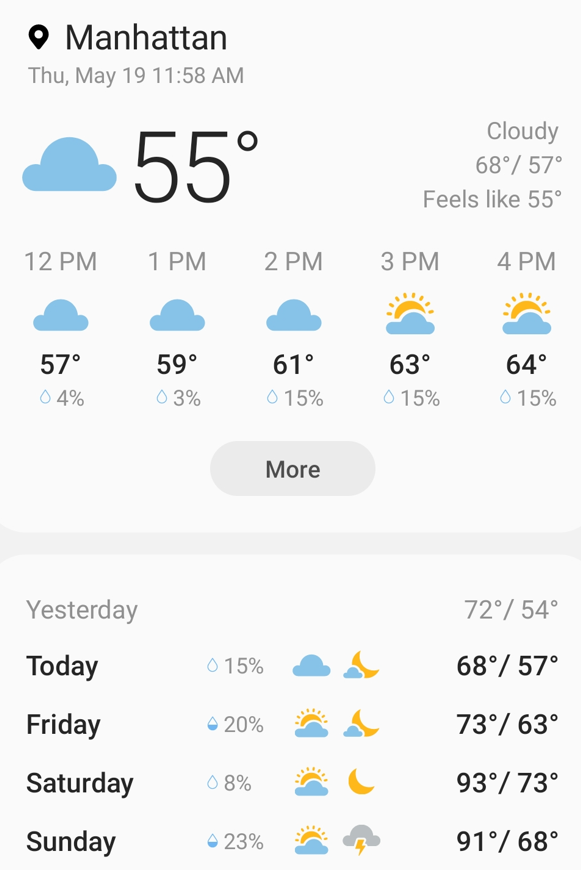The image showcases a weather app displayed on a tan or off-white background. In the upper left corner, there is a black GPS icon accompanied by the text "Manhattan." Beneath this, in gray print, it reads "Thursday, May 19th, 11:58 a.m."

The main weather information features a blue cloud icon indicating a temperature of 55°F. It states that it is "Cloudy, 68°F to 57°F" but feels like 55°F. The hourly forecast is as follows:

- 12 p.m.: 57°F with a blue cloud
- 1 p.m.: 59°F with a blue cloud
- 2 p.m.: 61°F with a blue cloud
- 3 p.m.: 63°F with a blue cloud and a hint of sun
- 4 p.m.: 64°F with a blue cloud and a hint of sun

Below these details, there is a "More" option. The extended forecast shows:

- Yesterday: 72°F to 54°F
- Today: 15% chance of rain, 68°F to 57°F, blue cloud during the day and a blue night sky
- Friday: 20% chance of rain, 73°F to 63°F, blue cloud with sun and moon icons
- Saturday: 8% chance of rain, 93°F to 73°F, blue cloud with sun and moon
- Sunday: 23% chance of rain, 91°F to 68°F, blue cloud with sun, followed by a storm cloud